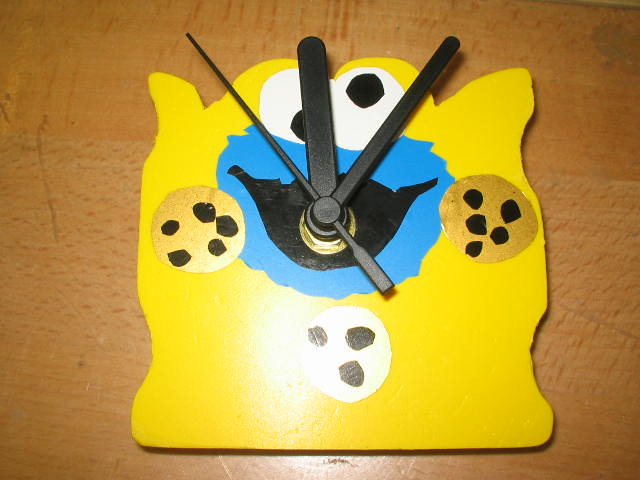This close-up photograph captures a uniquely crafted, homemade analog clock placed on a golden-brown wooden table. The clock is designed to resemble Cookie Monster, the beloved blue furry character with googly eyes and a big black mouth from which three black clock hands (seconds, minutes, and hours) emerge. The clock face is adorned with Cookie Monster's expressive eyes—one looking upward, the other downward—and is uniquely framed by a yellow irregularly shaped board that doubles as the clock's body. Instead of traditional numbers, there are three tan and dark brown chocolate chip cookies positioned at the 3, 6, and 9 o'clock positions. The entire image is brightly lit, with a notable reflection of light on the bottom portion of the clock, adding a vibrant touch to this whimsical timepiece.